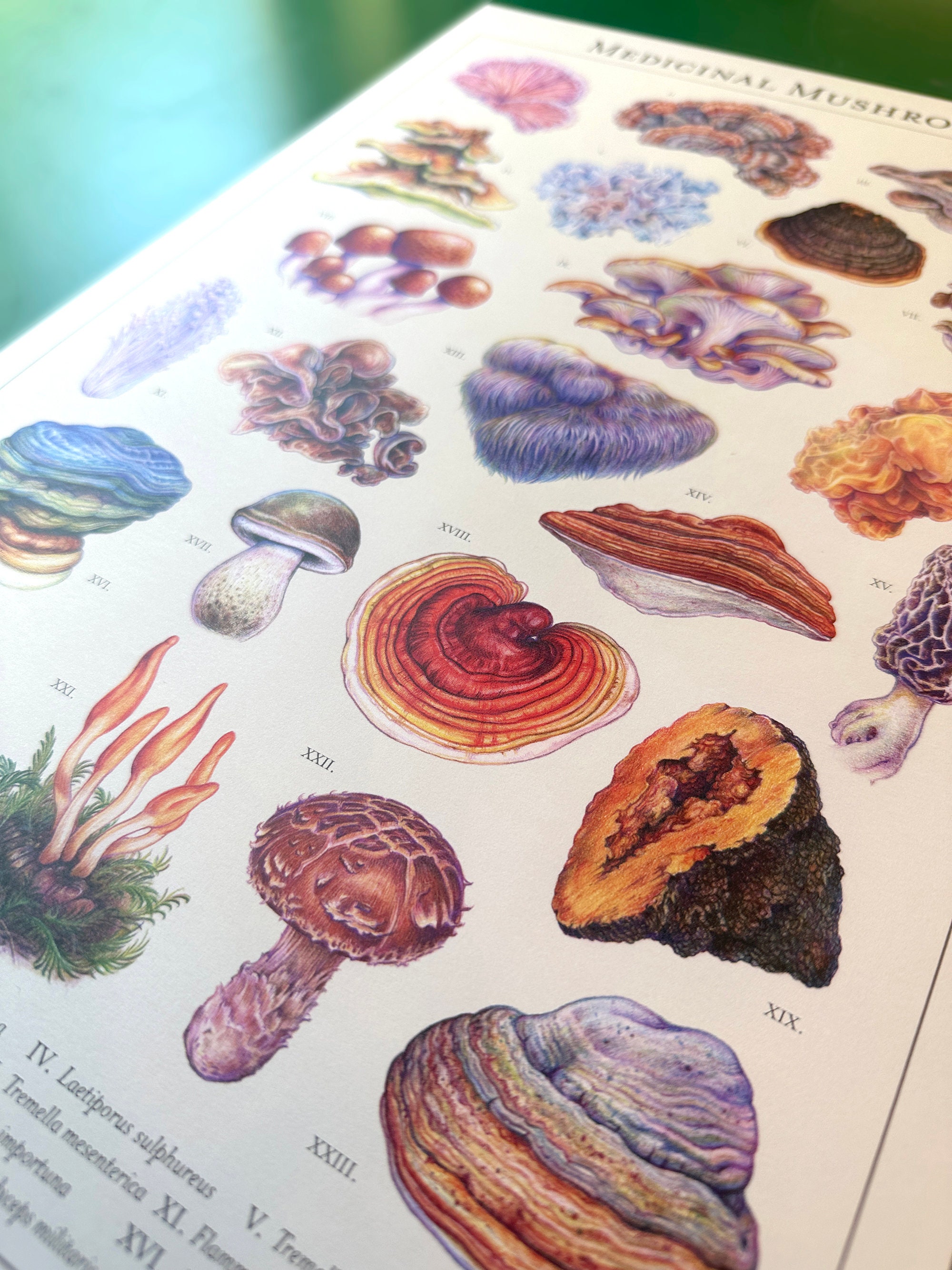The image appears to be a detailed photograph of a page from a biology textbook or a scientific reference book. The page is dedicated to “medicinal mushrooms,” prominently labeled at the top. The layout features between 20 to 25 intricately illustrated mushroom species, each rendered in a style that combines precise scientific detail with beautiful artistry. The illustrations vary in color, depicting a spectrum that includes white, brown, orange, blue, pink, yellow, and gray. Some mushrooms are shown as singular specimens with clear stems and caps, like the typical button mushroom, while others are depicted as clusters or mounds burgeoning amidst green vegetation.

The drawings are meticulously labeled with Roman numerals, ranging up to XVIII, adding an additional layer of scientific elegance. Although some labels are blurred, it's clear that the detailed scientific names are provided at the bottom of the page. The artistic quality of the illustrations is highlighted by both the vivid colors and the careful detailing of each mushroom's unique features, such as the shaggy textures and cross-sectional views revealing interior colors. This combination of scientific accuracy and artistic representation makes the page an informative and visually captivating section of the book.